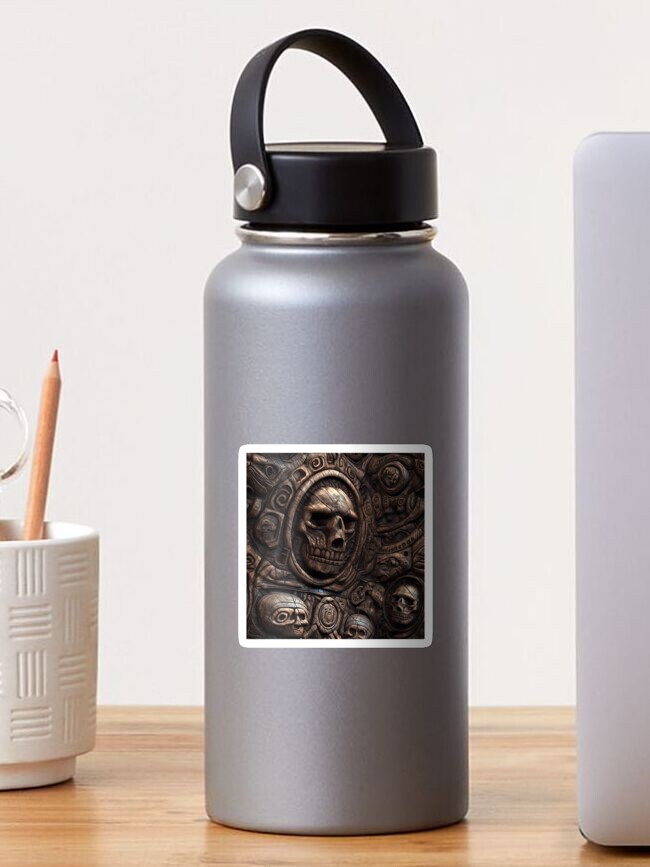This indoor photograph captures a scene on a light brown wooden table with a horizontal grain pattern and a plain white wall as the background. Central to the image is a tall, pewter-gray thermos with a black twist top and a black handle arching over it, secured by a circular silver metal piece. Adorning the center of the thermos is a square image outlined in white, displaying a detailed depiction of stone-carved skulls, featuring one large skull and three smaller ones. To the right of the thermos stands the partially visible back of a laptop case. To the left, there's a small white vase-like cup, embellished with patterned vertical lines, holding a pencil with its point up and a pair of silver scissors.